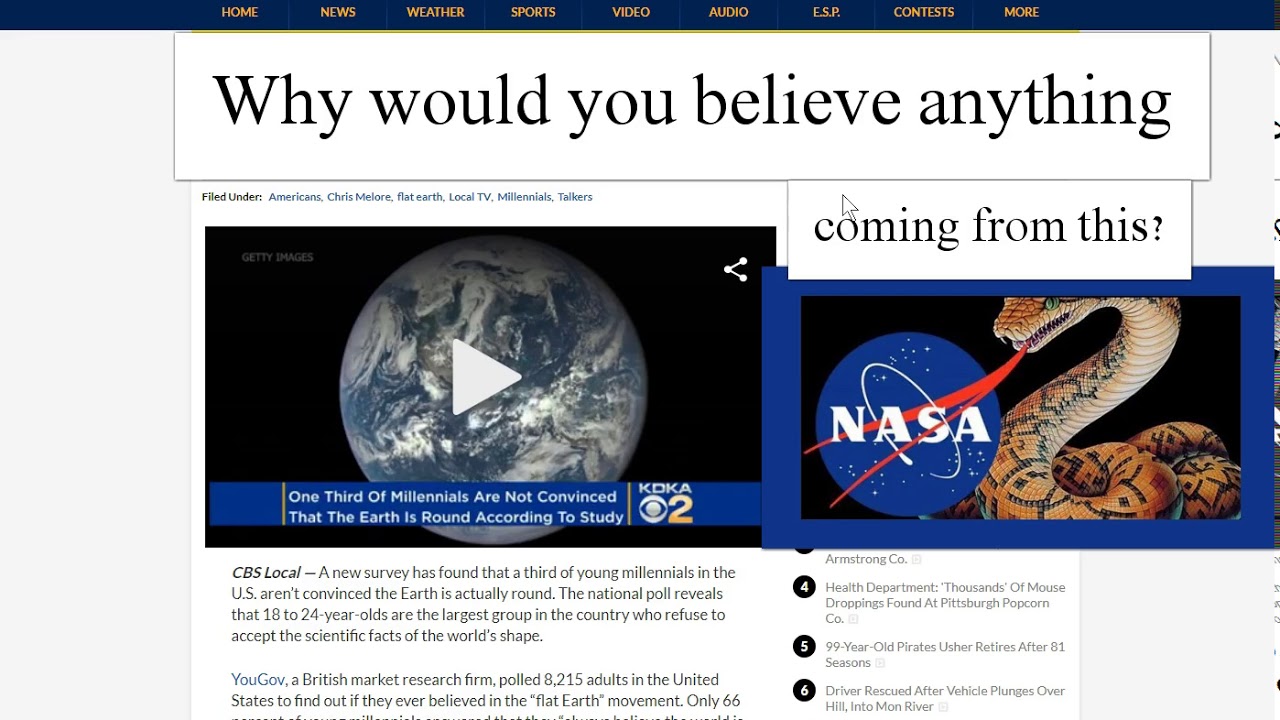The image depicts a webpage characterized by a navy blue navigation bar at the top, featuring various sections such as "Home," "News," "Weather," "Sports," "Video," "Audio," "ESP," "Contests," and "More," all written in yellow text. Below this bar, there is a prominent white box with the text "Why would you believe anything." 

Underneath this box, two side-by-side images are accompanied by descriptive text. On the left, there is an image of Earth from space with a headline stating, "One-third of millennials are not convinced that the Earth is round, according to a study." The caption explains that a survey by CBS Local found a significant portion of young millennials in the U.S., specifically those aged 18 to 24, doubt the Earth's roundness. This survey, conducted by the British market research firm YouGov, polled 8,215 students and revealed that only 66% accept the Earth as round, but the rest of the text is cut off.

To the right, there is another image featuring the NASA logo with a snake's tongue seemingly interacting with it. Below this image, several news items are listed along with corresponding numbers in bubbles: 
1. "4 - Health Department: Thousands of mouse droppings found at Pittsburgh Popcorn Co."
2. "5 - 99-year-old Pirates usher retires after 81 seasons."
3. "6 - Driver rescued after vehicle plunges over hill into Moon River."

This detailed layout offers a snapshot of various news and information sections available on the website.